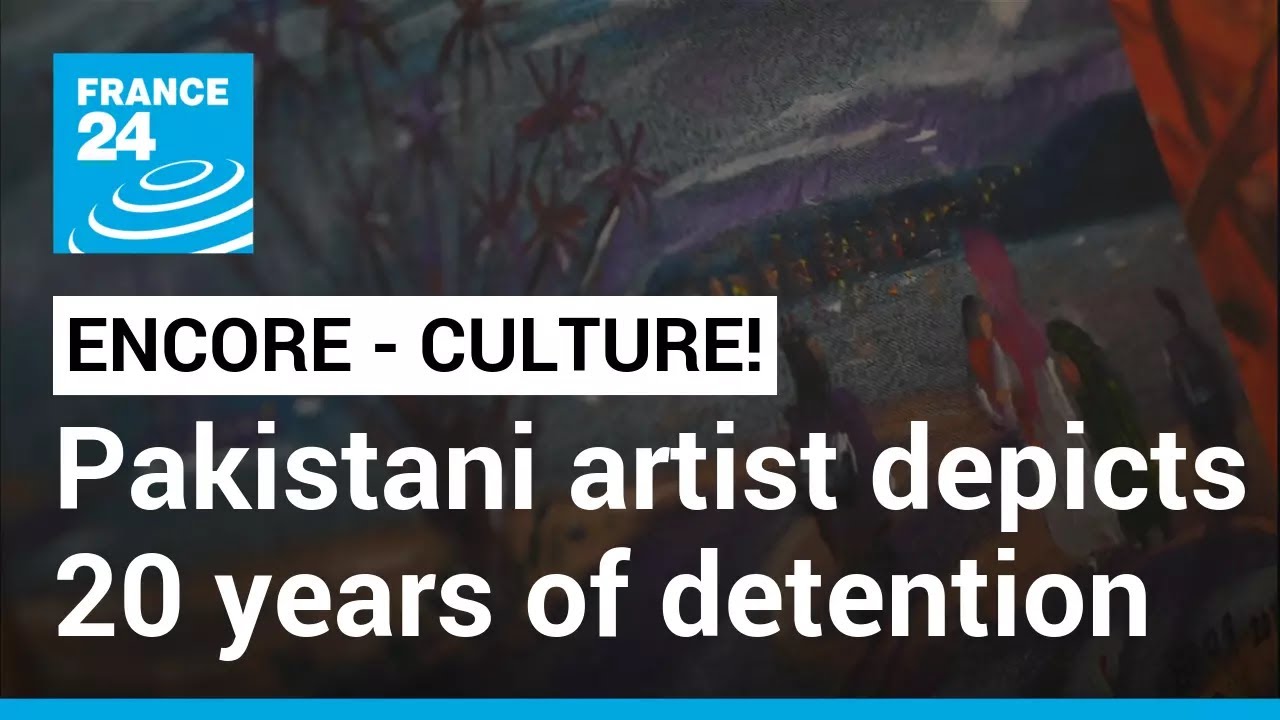This image, possibly from a news service segment on France 24, displays a blend of text and an illustration highlighting a Pakistani artist's work depicting 20 years of detention. Prominently featured in the top right is the blue, circular France 24 logo, with a white globe inside it. Directly below, in a white-bordered rectangle with black type, it states "Encore Culture!" and below that, in large white text, it says, "Pakistani artist depicts 20 years of detention." A blue stripe, matching the logo's color, runs along the bottom of the image.

In the background, there is a dark, evocative painting showing various figures wearing robes, set against a night scene with a dark purple sky and grey clouds. The artwork includes a line of people, possibly detainees, some dressed in red, with a tree and landscape elements subtly present. While the details of the painting are somewhat blurred, the overall atmosphere conveyed is somber, hinting at the gravity of long-term detention. This image likely serves as an advertisement for an art exhibit featuring the artist's poignant work.